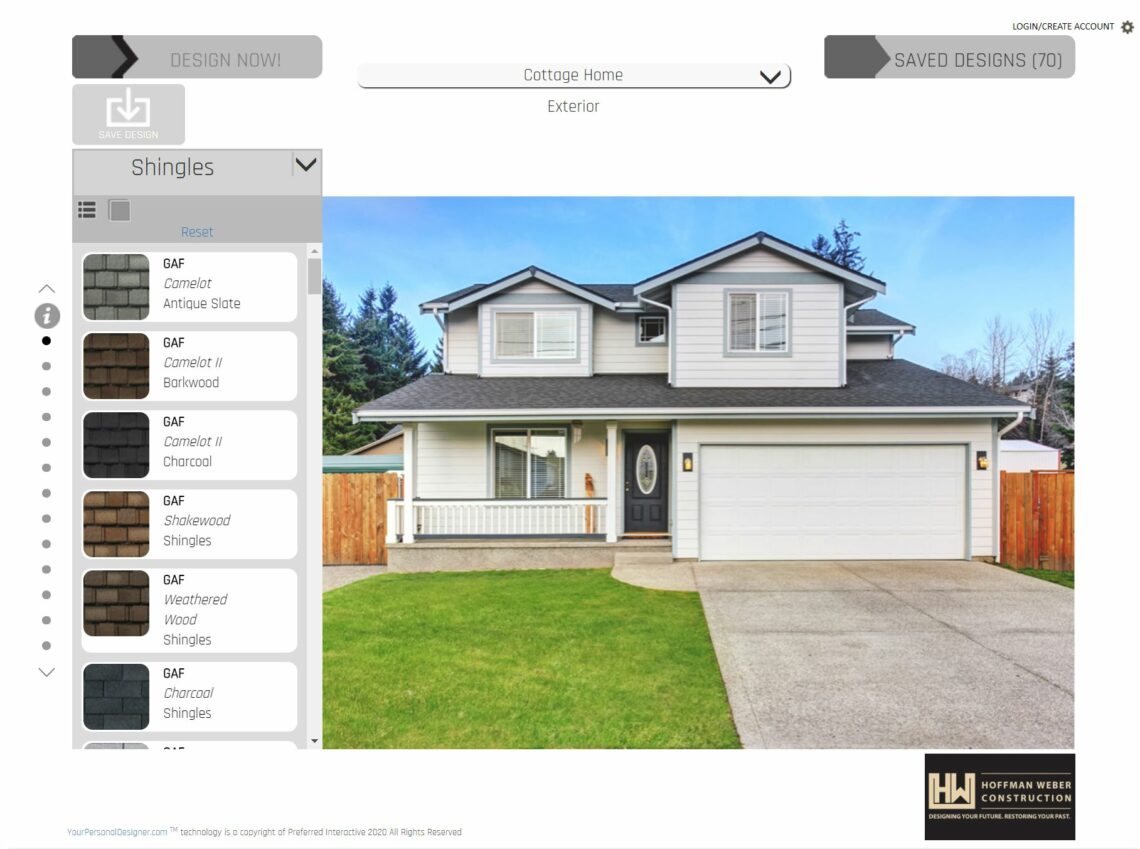This appears to be a screenshot of a website interface, likely from a design or construction platform. At the top of the image, on the left side, there is a gray box with a black arrow on its right side, and the text "Design Now" displayed prominently. To the right of this box, there is another gray box with a gray arrow extending towards the end of the bar, labeled "Saved Designs (70)."

Between these two boxes, there is a drop-down menu labeled "Cottage Homes," accompanied by a white bar and a downward-facing arrow. Below this, there is another label that reads "Exterior." Directly underneath the "Design Now" box on the left, there is a gray box with a downward-pointing arrow and the text "Save Design."

Further down, there's a menu named "Shingles," offering various options for shingle selections. 

The main body of the image on the right side features a picture of a white house with a gray roof. At the bottom of the screen, there is white space with some text located at the bottom left. On the bottom right, there is a black box containing a logo and the text "Hoffman Weber Construction" with additional text underneath it.